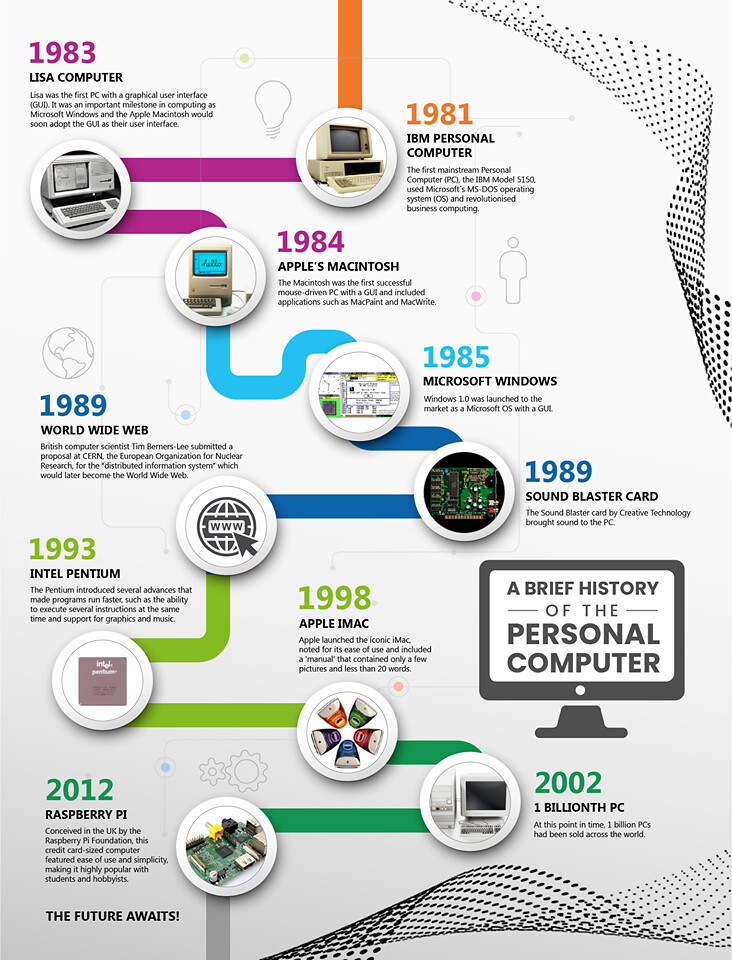This image features a detailed, rectangular flyer that serves as a timeline of the personal computer's history. At the top, it begins with an orange circle highlighting the 1981 IBM Personal Computer, showing a picture of it. A purple line then leads to the 1983 Lisa Computer, followed by another purple line to the 1984 Apple Macintosh, each accompanied by their respective images. Transitioning to light blue, the timeline moves to the 1985 Microsoft Windows, and then to a darker blue for the 1989 Sound Blaster card, which is depicted with an image of a mechanical card or chip. The timeline continues in blue to mark the introduction of the World Wide Web in 1989. 

In 1993, a green section denotes the release of the Intel Pentium, and in 1998, another green line leads to the Apple iMac. A darker green circle marks the milestone of 1 billion PCs in 2002. The final highlighted event in the timeline is the 2012 release of the Raspberry Pi, also in green. All these events are connected by lines of varying colors, with each year and its technological milestone marked within circles that include images representing the event. 

Towards the bottom-right of the flyer, an image of a computer monitor displays the text "A Brief History of Personal Computers." The timeline concludes with a black text line that reads, "The Future Awaits."